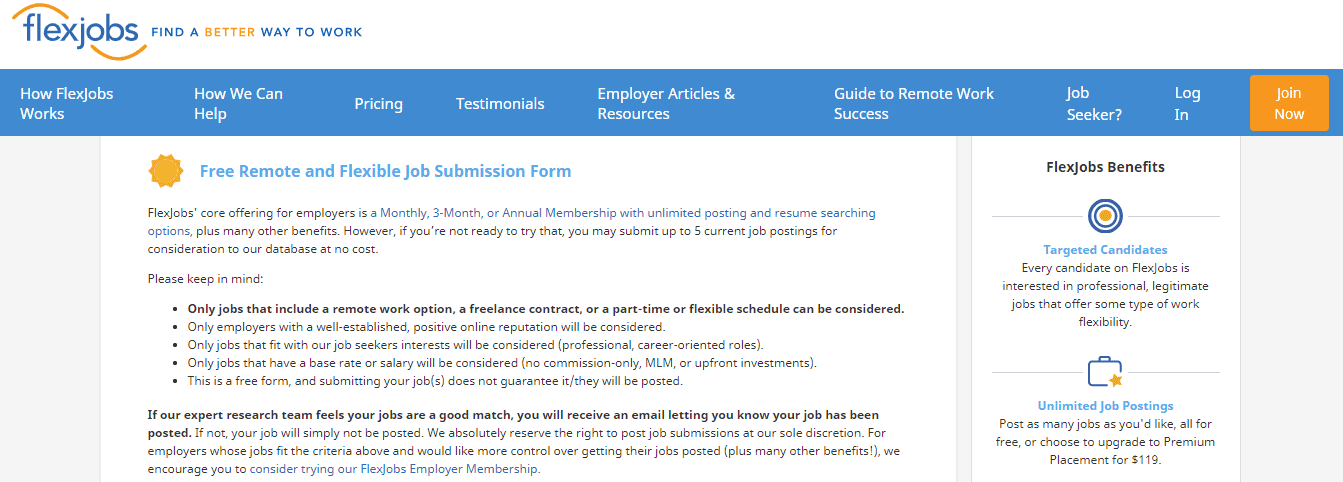The image features the homepage of the website Flexjobs. Dominant on the page is the company name "Flexjobs," spelled in blue letters with half of an orange infinity swirl integrated into the design. It’s set against a clean white background. Below the logo is the company slogan, "Find a Better Way to Work," where the word "better" is highlighted in orange to match the infinity swirl.

The navigation bar, colored in blue with white text, offers sections on pricing, testimonials, employee articles and resources. It serves as a comprehensive guide for both employers looking to place ads for remote positions, and job seekers searching for remote work opportunities. The homepage provides clear instructions in black text on how to use the site efficiently, either by logging in or joining as a new user.

The page is designed to inform visitors about the paid services offered by Flexjobs, showcasing a structured layout where potential users can easily learn how to join or utilize the website’s features.